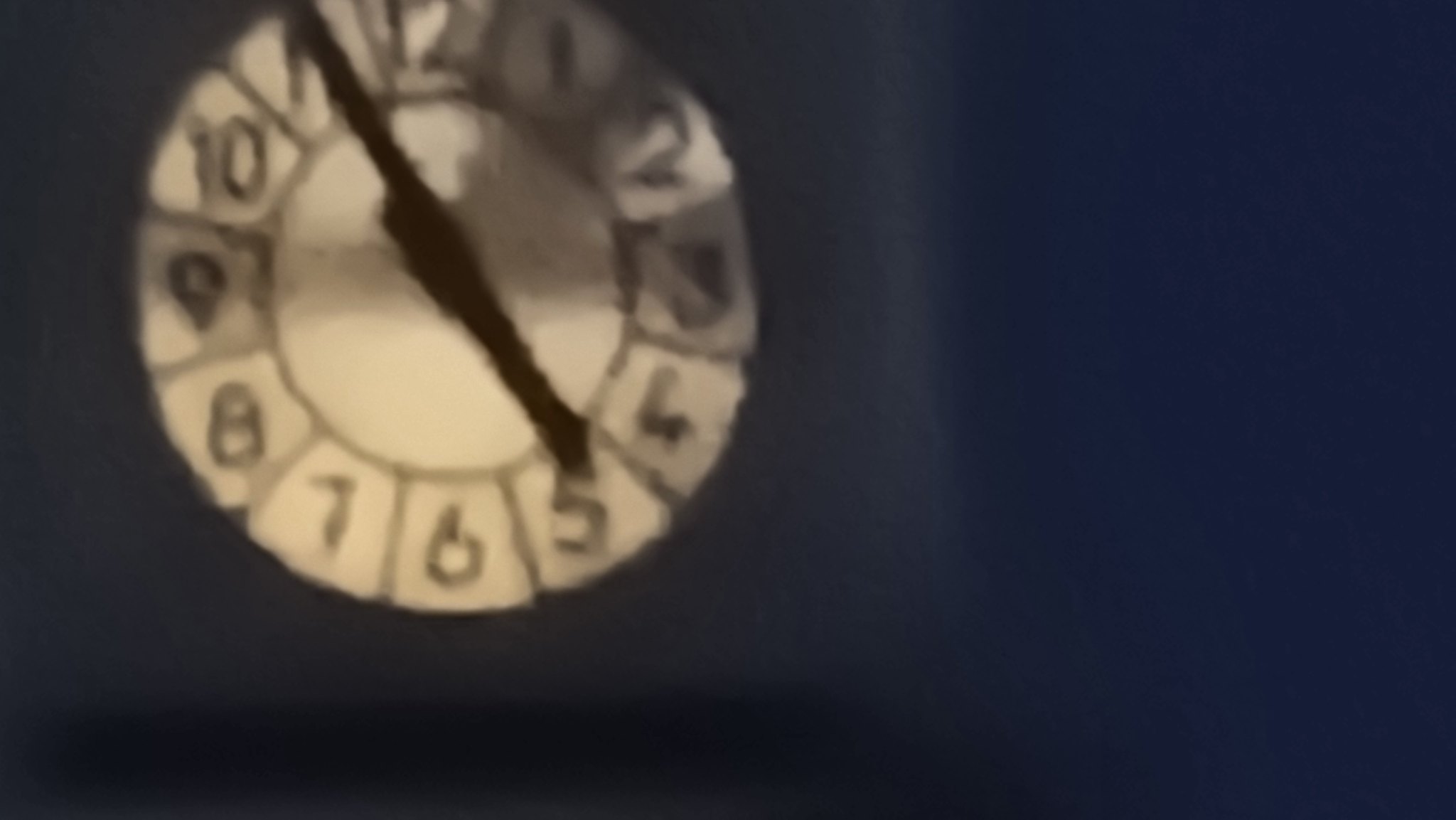The image is an illustration of a clock embedded into a two-tone blue wall, with a darker royal blue background and a lighter blue surrounding the clock face. The white, circular clock face features regular numbers (1 through 12) in black, each enclosed in its own individual square, creating a flower-like pattern with the central white circle acting as the "core" and the numbered squares as "petals." The clock hands are solid black, with the minute hand pointing to the 11 and the hour hand to the 5, indicating the time as 4:55. The clock appears to be a training aid rather than a functional timepiece. The setting is dark overall, adding to the glowing prominence of the clock’s golden shade, further highlighted by subtle light accents around its face.